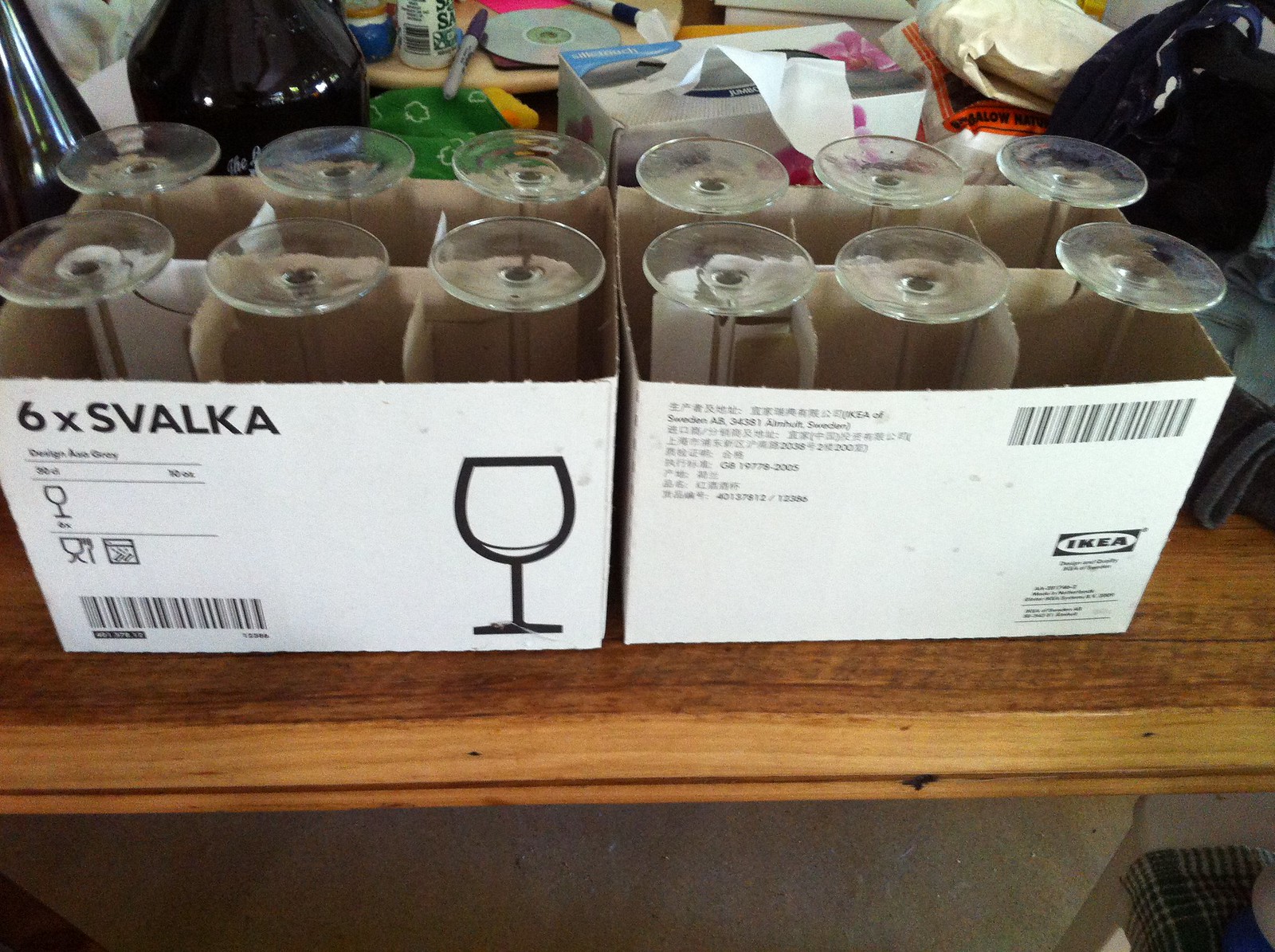In this photograph, a wooden table, seemingly unfinished, serves as the platform for two white cardboard boxes of wine glasses from Ikea. Each box contains six identical, upside-down wine glasses made of clear glass, with their stems pointing upward. The boxes are labeled with bold black text reading "6XSVALKA," accompanied by the Ikea logo and additional, smaller, unreadable text. The scene is cluttered with various items in the background, including a tissue box with a tissue protruding, a compact disc, several Sharpies, rags, and other miscellaneous cloths, creating an impression of disarray, possibly hinting at a garage sale or hoarding scenario.